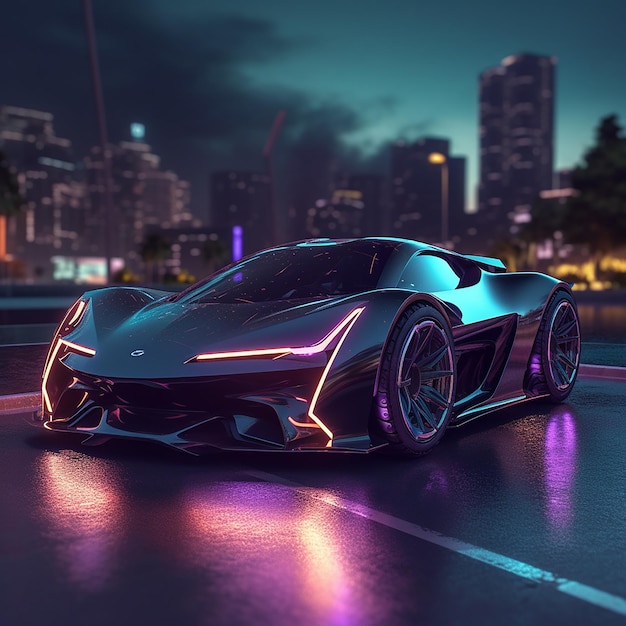The image features a sleek, futuristic electric concept car, blending design elements reminiscent of a Lamborghini and the Batmobile. Its body is curvy and ultra-modern, crafted from a shiny blue metal without visible seams for the doors. The car, situated in a dimly-lit paved parking lot with white diagonal stripes, is highlighted by reflective pinkish-purple lights on its tires and below it on the asphalt. Instead of conventional headlights, thin, illuminated lines run across the front, adding to its avant-garde appearance. A cityscape forms the backdrop, with tall skyscrapers lit up against a late-evening sky. To the right, the sky is a medium blue, while to the left, ominous black clouds are creeping over. The overall scene is infused with ambient purple and yellow lights, contributing to the image's otherworldly, digital aesthetic.